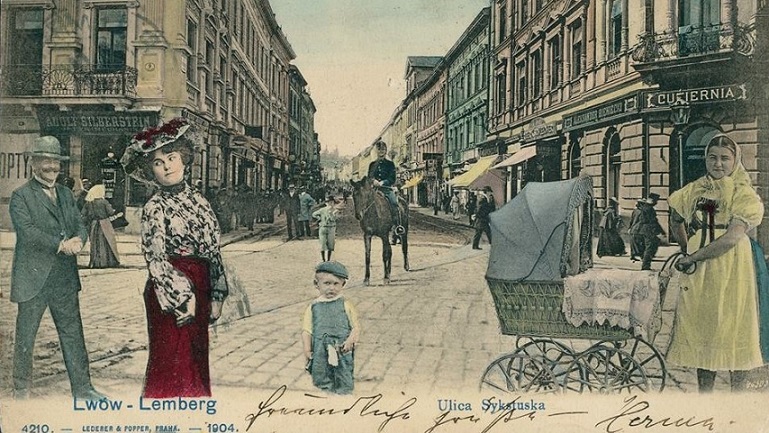A charmingly colorized image from a 1904 photograph postcard captures a bustling European city street, identified as Lemberg (L.W.O.W.), now Lviv in Ukraine. The scene portrays cobblestone streets lined with three-story buildings, featuring shops on the ground level and apartments above. Distinct blues and yellows add a touch of life to the originally black-and-white scene. On the left, a man dressed in a late 1800s style suit and hat smiles with a big mustache. In front of him, a woman in a maroon skirt and intricate black flowery shirt dons a fancy hat, embodying a graceful Victorian style. Nearby, a small child in adorable overalls and a beret-type hat strolls along. To the right, another young woman in a muted yellow dress pushes an old-fashioned baby carriage with large spoked wheels and a hooded cover. Adding to the historical ambiance, a police officer on horseback patrols the street, marking the era before automobiles. The updated colors and the postcard's attempt to achieve a three-dimensional effect blend seamlessly, furthering the timeless European charm of this vibrant early 20th-century cityscape.